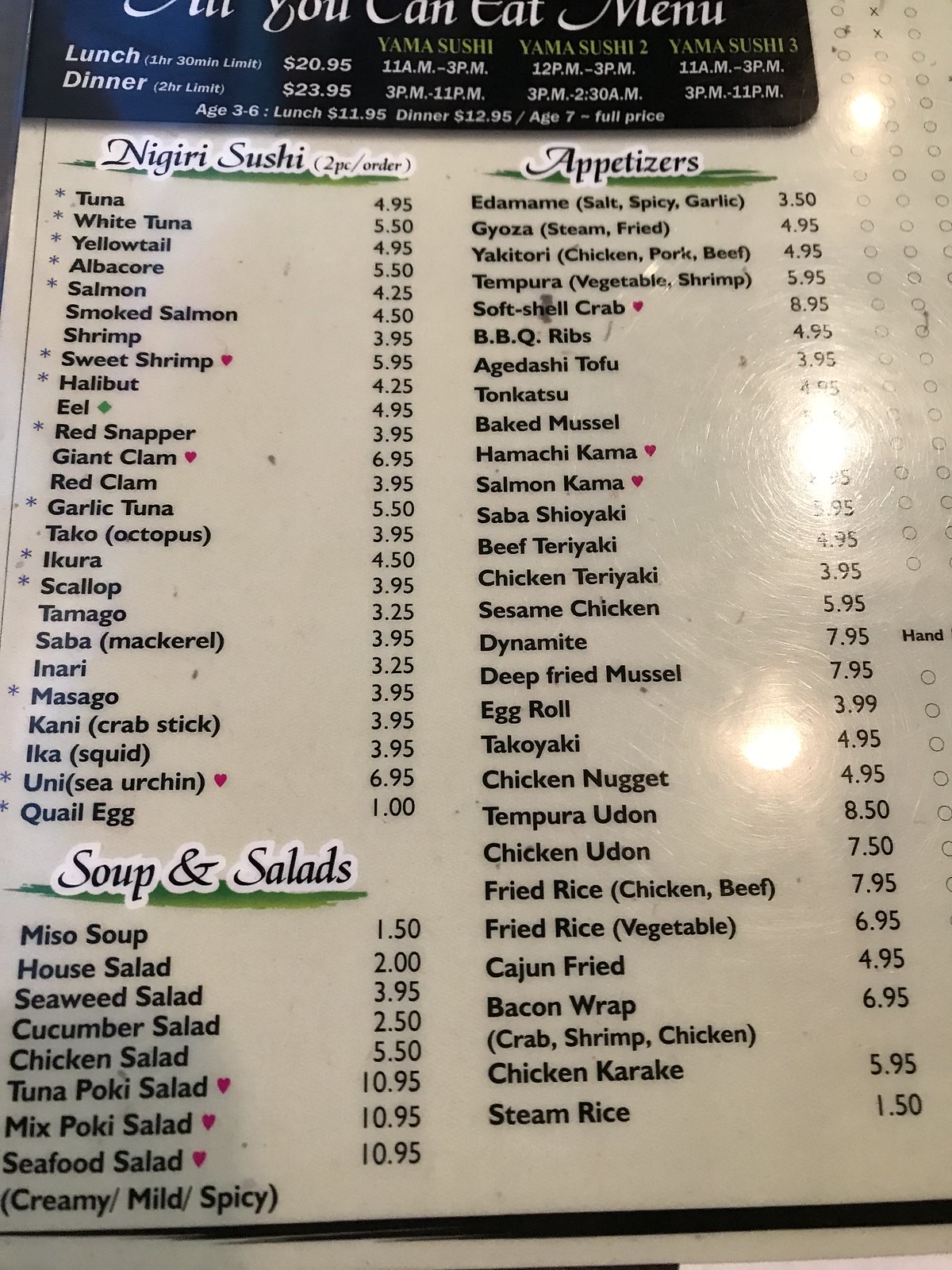The image features a well-lit restaurant menu printed on white laminated plastic. The glossy surface of the menu reflects the glow of three overhead lights, adding a subtle shine. The text on the menu is in English, detailing a variety of Japanese cuisine options. 

Under the sushi section, diners can find nigiri sushi available in two-piece orders. Specific offerings include Tuna Nigiri ($4.95), White Tuna Nigiri ($5.50), and Yellowtail Nigiri ($4.95). A variety of other tuna-based dishes are also present. In the Soups and Salads section, notable items are Miso Soup priced at $1.50, a House Salad for $2.00, and Seaweed Salad at $3.95, among other selections. 

To the right, the Appetizers section lists several tantalizing choices, such as Edamame prepared with salt, spicy, or garlic variations for $3.50, and Gyoza, either steamed or fried, for $4.95. The menu boasts an extensive range of appetizers to cater to different tastes.